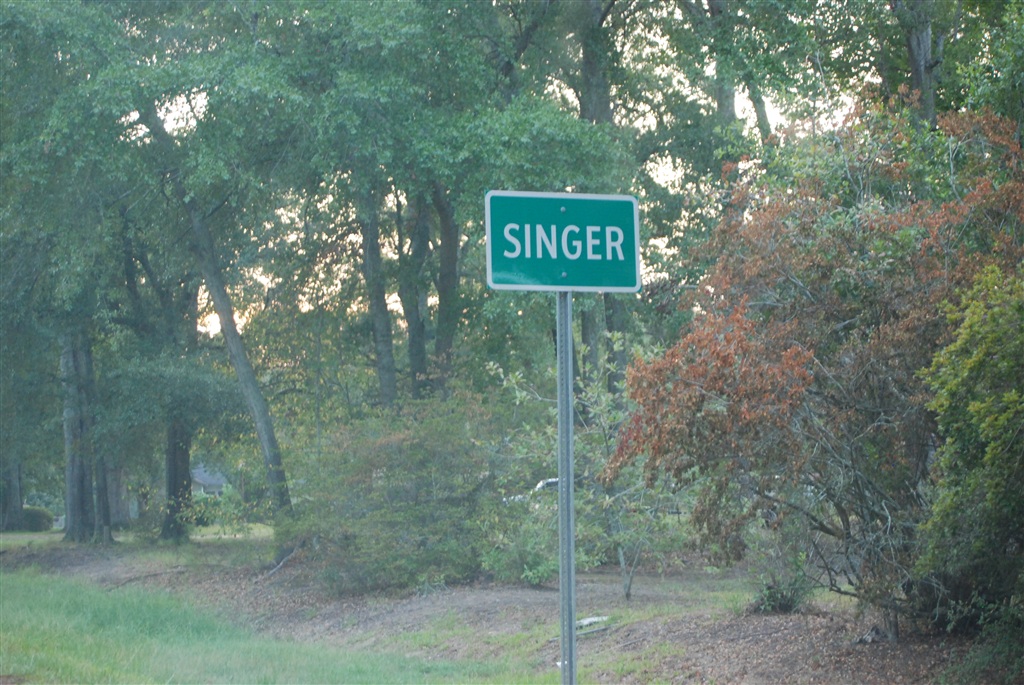This landscape-oriented photograph captures a scenic roadside view, seemingly taken from the vantage point of a passenger in a moving vehicle. The scene showcases a lush backdrop of green trees, with hints of reddish-orange and yellow foliage on smaller bushes towards the right side, indicating the turn of the seasons. At the center of the frame stands a signpost bearing a small green highway sign with the word "Singer" inscribed in white letters. The sign is mounted on a sturdy green metal plate. The golden hues of the light filtering through the trees suggest that this photograph was taken late in the day, imparting a warm, tranquil atmosphere to the composition.